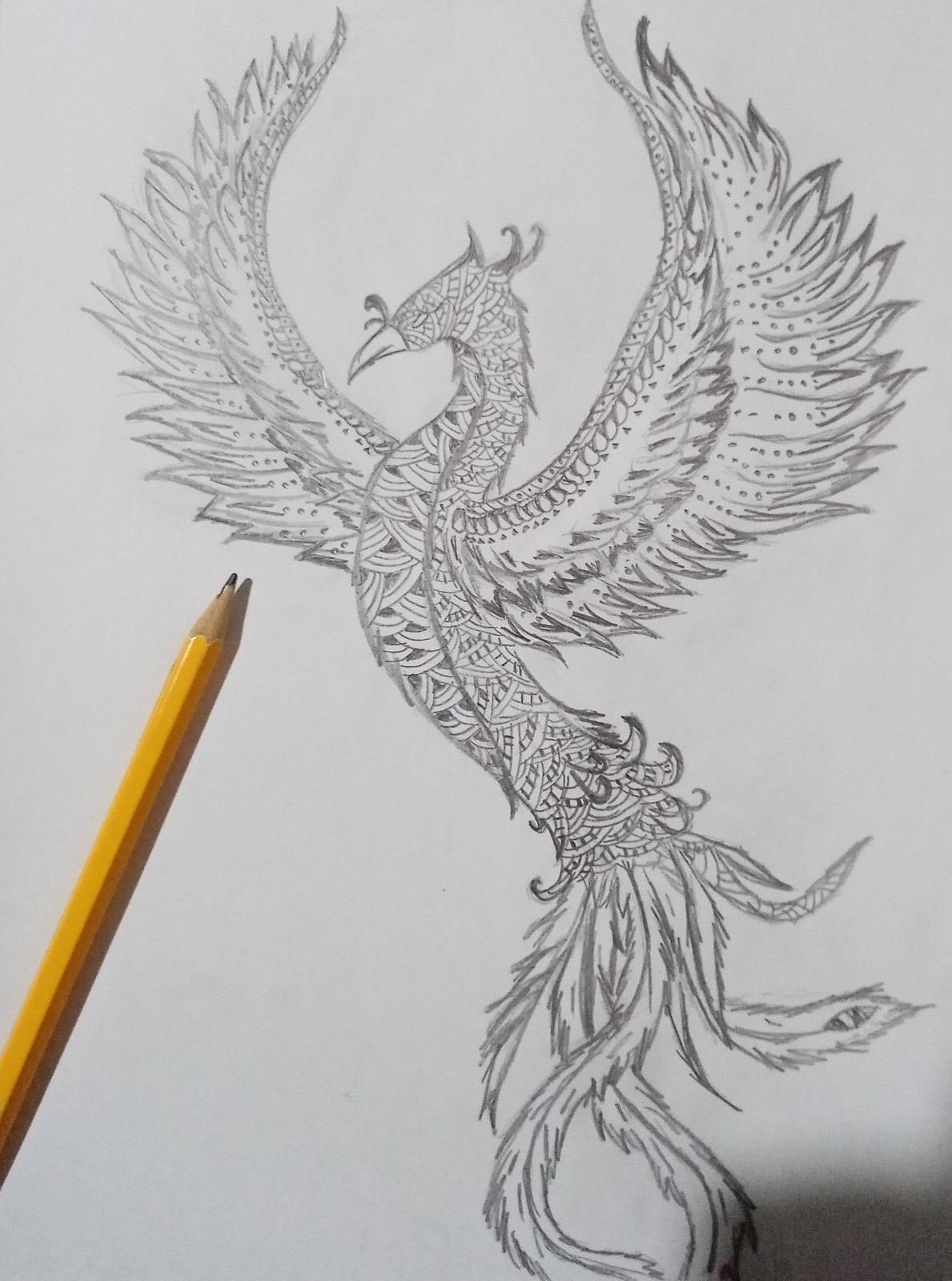This is a meticulously crafted, highly stylized pencil drawing of a dragon, designed with remarkable intricacy and attention to detail. The dragon, or fire-breathing creature, features expansive, elegantly detailed wings adorned with stylized feathers. Its robust chest and central body are elaborately embellished with a variety of intricate shapes and patterns, including curls, dots, squares, and rectangles. Additionally, small beak-like forms are interwoven within these motifs, adding to the complexity of the design. The dragon’s beak is firmly shut, and no facial expressions are visible, emphasizing an air of mystique. Despite the lack of shading or depth, the image captivates with its decorative precision and the harmonious arrangement of stylized elements. The exact type of pencil used by the artist remains indeterminate, yet the overall execution showcases a superb mastery of line work and decorative artistry.